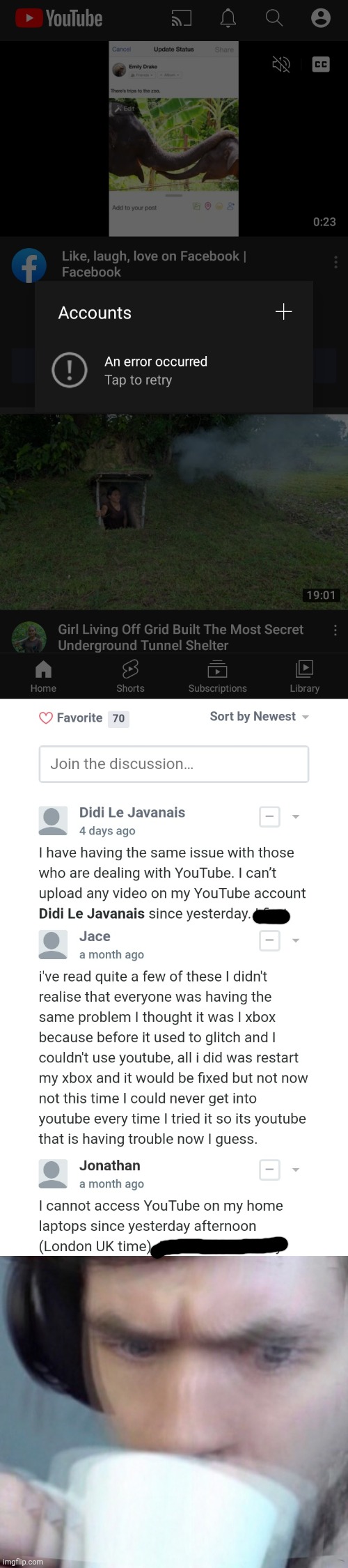### Descriptive Caption for the Image Collection

This image collection consists of several screenshots depicting issues users are experiencing with the YouTube mobile application and a related discussion thread from a different app. The first screenshot highlights the YouTube mobile app, featuring a darkened background with a few video thumbnails. A prominent dark gray pop-up occupies the center, displaying "Accounts" in white text at the top left, with a plus sign icon on the top right. Below this, there's a light gray circular ‘donut’ icon with an exclamation mark and the message, "An error occurred," followed by light gray text instructing users to "Tap to retry."

The second screenshot captures a discussion thread interface on a mobile application, set against a white background. At the top, there's a text box outlined in light gray with placeholder text, "Join the discussion..." in light gray. Below this, three user messages are shown.

1. The first message reads: "I having the same issue with those who are dealing with YouTube. I can’t upload any video on my YouTube account. Didi Lejavenais (J-A-V-A-N-A-I-S), since yesterday." Some text to the right is blacked out.
   
2. The second message from Jace says: "I’ve read quite a few of these. I didn’t realize that everyone is having the same problem. I thought it was my Xbox because before it used to glitch and I couldn't use YouTube. All I did was restart my Xbox and it would be fixed, but not now, not this time. I could never get into YouTube every time I tried it. So it’s YouTube that is having trouble now, I guess."

3. The third message from Jonathan states: "I cannot access YouTube on my home laptops since yesterday afternoon (London, UK time)." Additional text to the right is blacked out.

The final screenshot captures an image of a man wearing large black headphones and drinking from a white cup. The photo is intentionally blurred, creating an effect akin to double vision, highlighting the disorientation and frustration users might feel due to the YouTube issues.

This collection of screenshots provides a detailed snapshot of ongoing technical problems faced by users on the YouTube platform and their shared experiences in troubleshooting these issues.